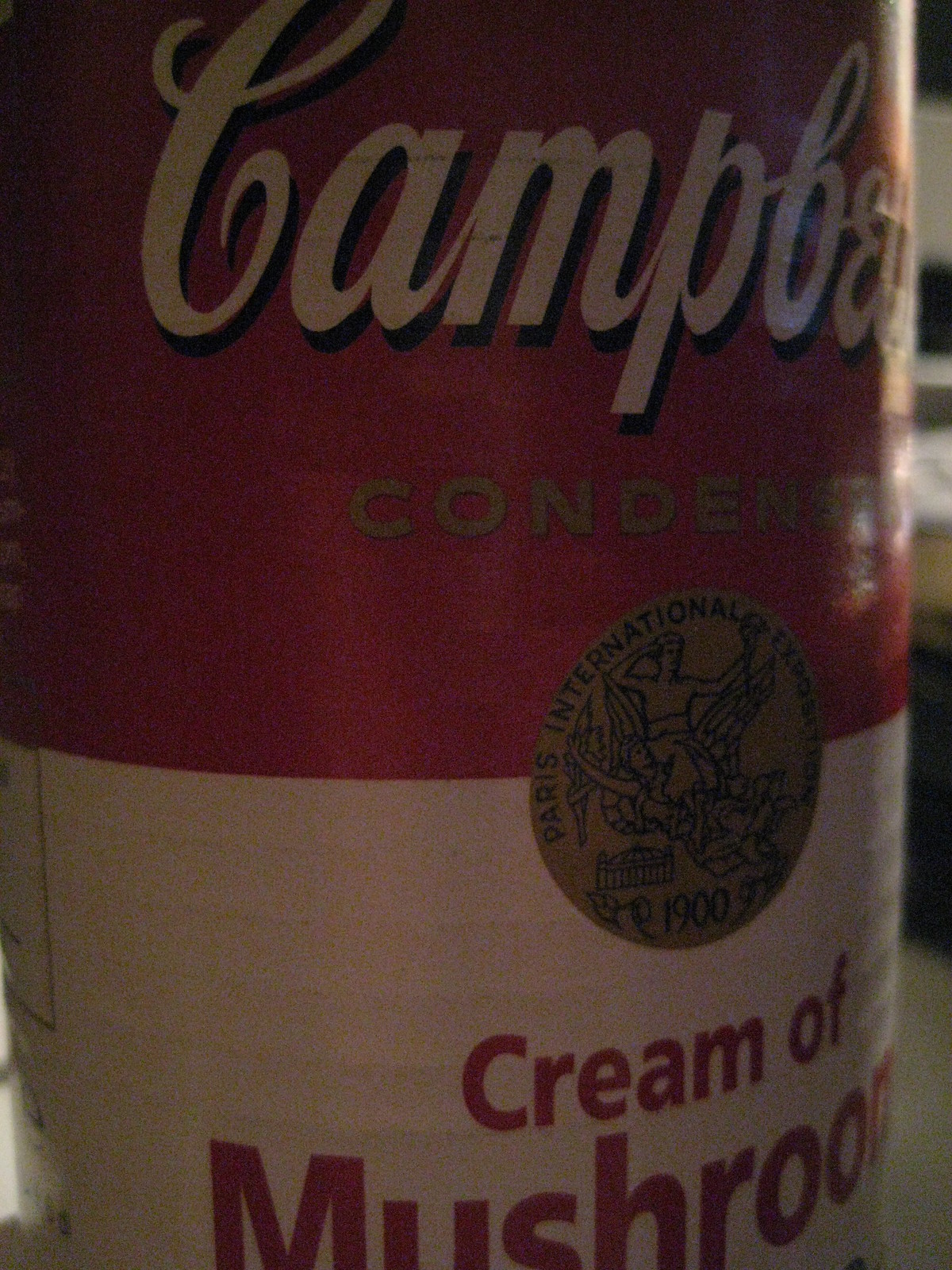This close-up photograph showcases a can of Campbell's Condensed Cream of Mushroom Soup prominently displayed on a white kitchen counter. The iconic can is divided into two main color sections: the top half is a vibrant red, and the bottom half is a crisp white. In the red section at the top, the Campbell's logo is elegantly written in white cursive script. Just below, a gold medallion featuring a Greek-inspired man seated on an elaborate throne adds a touch of classic detail. The word "Condensed," also in gold, is positioned beneath the medallion. The white portion of the can displays the product name, "Cream of Mushroom Soup," in bold red letters. The background subtly reveals elements of a kitchen, grounding the can in a domestic setting.